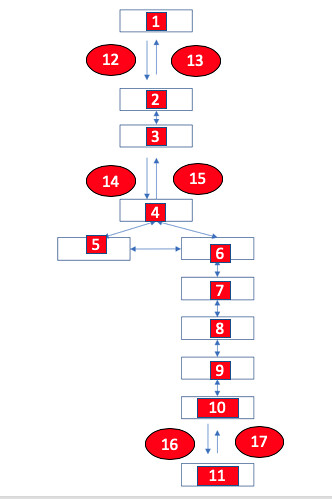The image portrays a digitally created diagram with a pristine white background. A sequence of 17 rectangular boxes, numbered from 1 to 17, is systematically arranged with their longer sides oriented horizontally. Each box is delineated with a medium blue outline and is empty within.

Inside each rectangle, there is a small, thin black-outlined box filled with a vibrant red color, featuring a white numeral at its center to indicate the sequence. Connectivity between these boxes is illustrated using directional arrows, highlighting the interrelationships.

At the top of the diagram, Box 1 initiates the sequence. Arrows project from Box 1 in two directions: one arrow directing towards Box 2 below and another looping back from Box 2 to Box 1. Flanking these arrows, positioned to the left and right, are two horizontal ovals numbered 12 and 13 respectively.

Proceeding downward, Box 2 connects to Box 3 with another set of arrows, which is mirrored in the pattern seen between Boxes 3 and 4. In the space between Boxes 3 and 4, the sequence includes ovals numbered 14 and 15.

The layout continues in a similar structured fashion, culminating with Box 11 at the bottom right corner of the image. The intricate network of numbered boxes and directional arrows together form an elaborate mapping of connections, ensuring a coherent flow of information throughout the diagram.